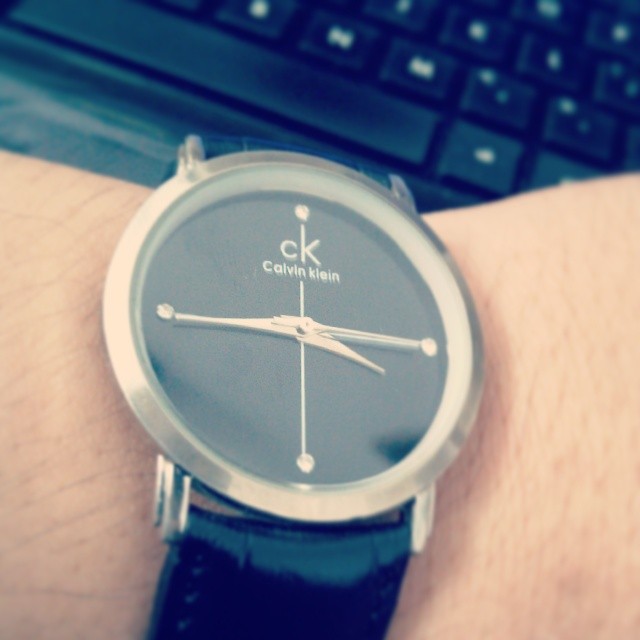The photograph showcases a close-up of a wrist adorned with a sophisticated wristwatch. The watch features a black leather strap that seamlessly connects to a sleek silver metal housing, possibly made of silver or stainless steel. The watch face is a striking black, prominently displaying the "CK Calvin Klein" logo. Notably, the 12, 3, 6, and 9 o'clock positions on the dial are marked by small stones, which could be diamonds or another type of gemstone, adding a touch of elegance. In the background, a black keyboard is visible, suggesting that the photo was taken near a computer workstation.